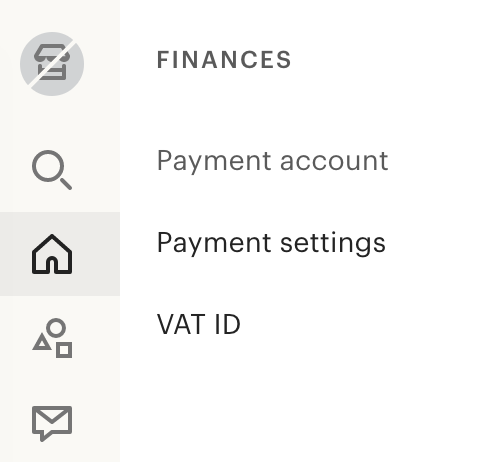In this image, set against a plain white background, there is a simple and large vertical navigation bar on the left side, featuring a slightly tan and gray color scheme. The navigation bar contains various icons, each paired with a corresponding label in capitalized gray text. 

Starting from the top, the first icon is a house or building within a gray circle, with a diagonal white line dividing it from the lower left to the upper right. To its right, the label reads "FINANCES." The second icon below this is a magnifying glass, with the label "PAYMENT ACCOUNT" beside it. The third icon is a home symbol, indicating "PAYMENT SETTINGS" to its right. 

Further down, there is an icon displaying three geometric shapes—a small gray circle, a rectangle, and a triangle—inside a box, with the label "VAT ID" in black text next to it. The final icon located at the bottom left corner is an envelope.

This navigation bar appears to serve as an interface for managing various financial and account settings, organizing its options clearly with intuitive icons and concise text labels.